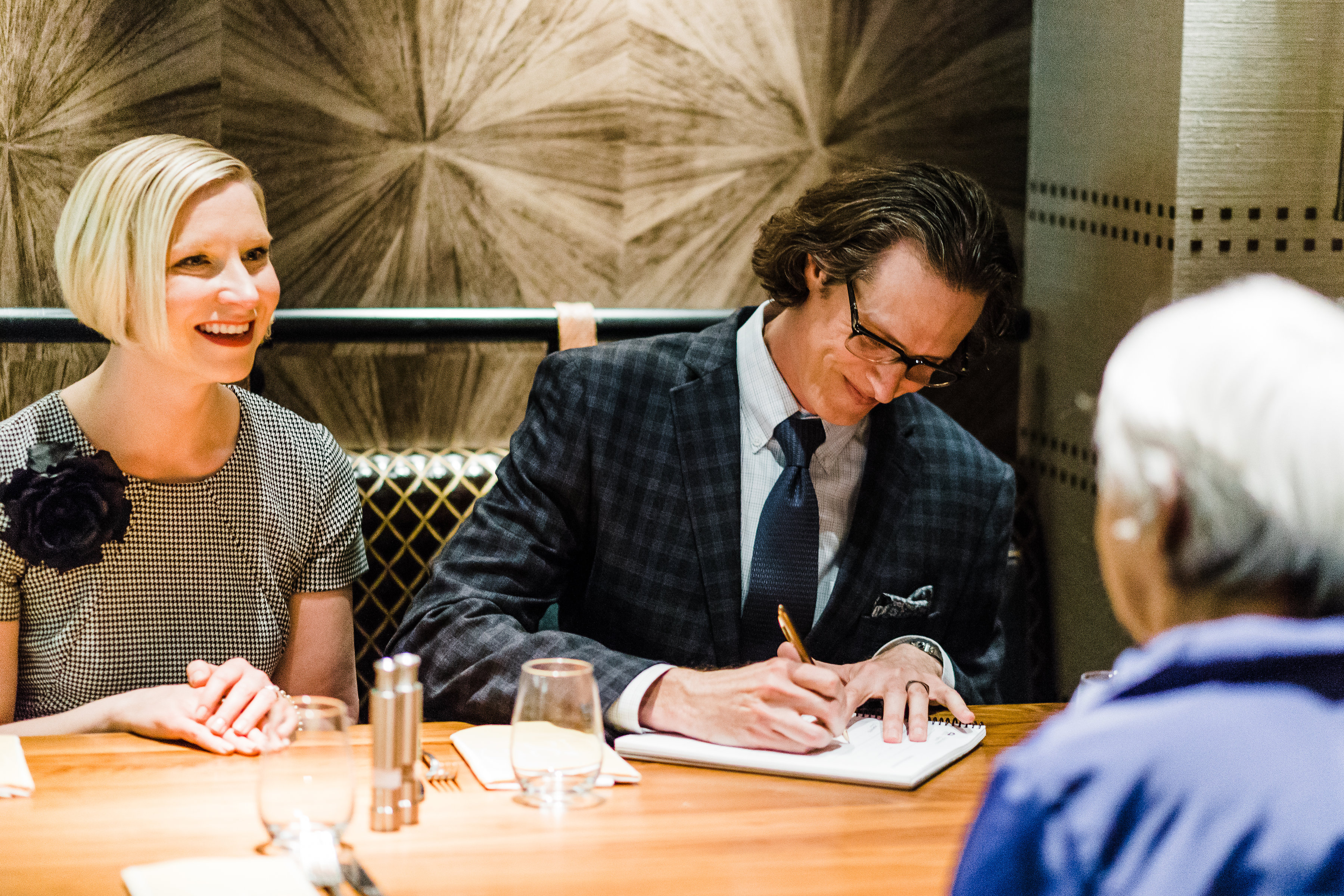In a cozy, warmly lit indoor setting with abstract gray-brown wallpaper, three individuals are seated at a light brown wooden desk that suggests a restaurant ambiance. On the left is a blonde-haired woman with a winning smile, her hair parted right to left and just touching her jawline. She is dressed in a gray and white dotted shirt adorned with a black blotch on her left shoulder, and her hands rest gently on the table before her. Across from her, to the right, sits a man immersed in his tablet. His dark gray hair falls to mid-shoulder, swept back neatly behind his black glasses. He dons a white suit with blue and black stripes over a light blue shirt and a matching blue tie. A gold pen in one hand and the other hand on the tablet, he appears focused on his writings. Between them, an empty clear glass graces the table, hinting at a recent or anticipated refreshment. In the out-of-focus lower right corner, another figure with gray hair, clad in a blue jacket with a collar, subtly completes the scene. The photograph captures a moment shared amidst details of their attire and surroundings.